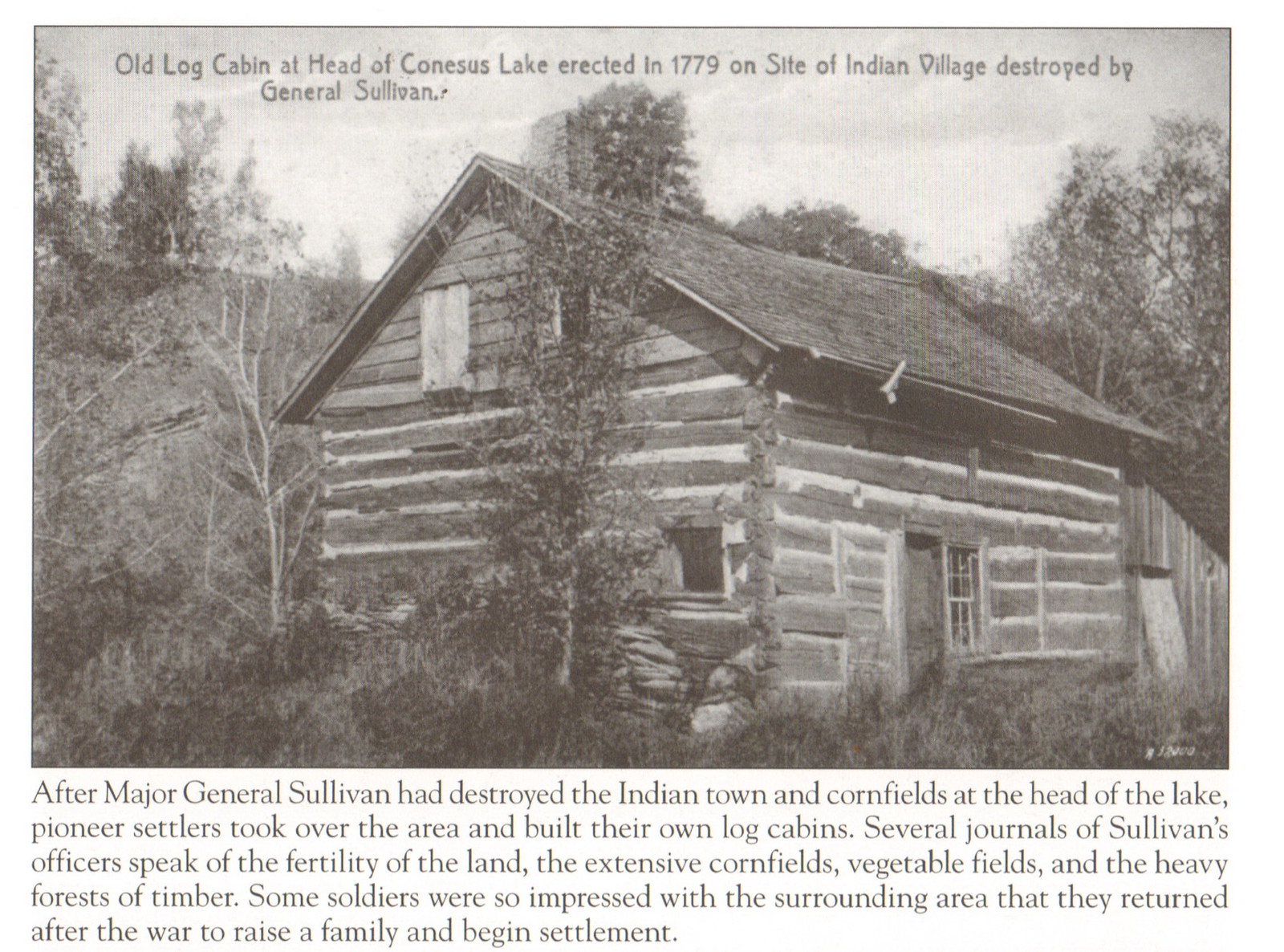The black and white image depicts an old log cabin, erected in 1779 at the head of Canisius Lake, on the site of an Indian village destroyed by General Sullivan. The cabin, constructed with logs and mud, appears uninhabited and in a state of disrepair, surrounded by trees and overgrown weeds. Notably, some windows are boarded up while others are not, and they do not sit flush within their frames. The roof, an A-frame style with shingles, also shows significant deterioration. An inscription at the top of the image details its historical context, mentioning the land's transformation post-Sullivan's campaign. Underneath the image, a paragraph elaborates on how pioneer settlers, attracted by the land's fertility, cornfields, vegetable fields, and heavy forests, built their own log cabins. Several soldiers who served with Sullivan were so captivated by the area's richness that they returned after the war to establish settlements and raise families.